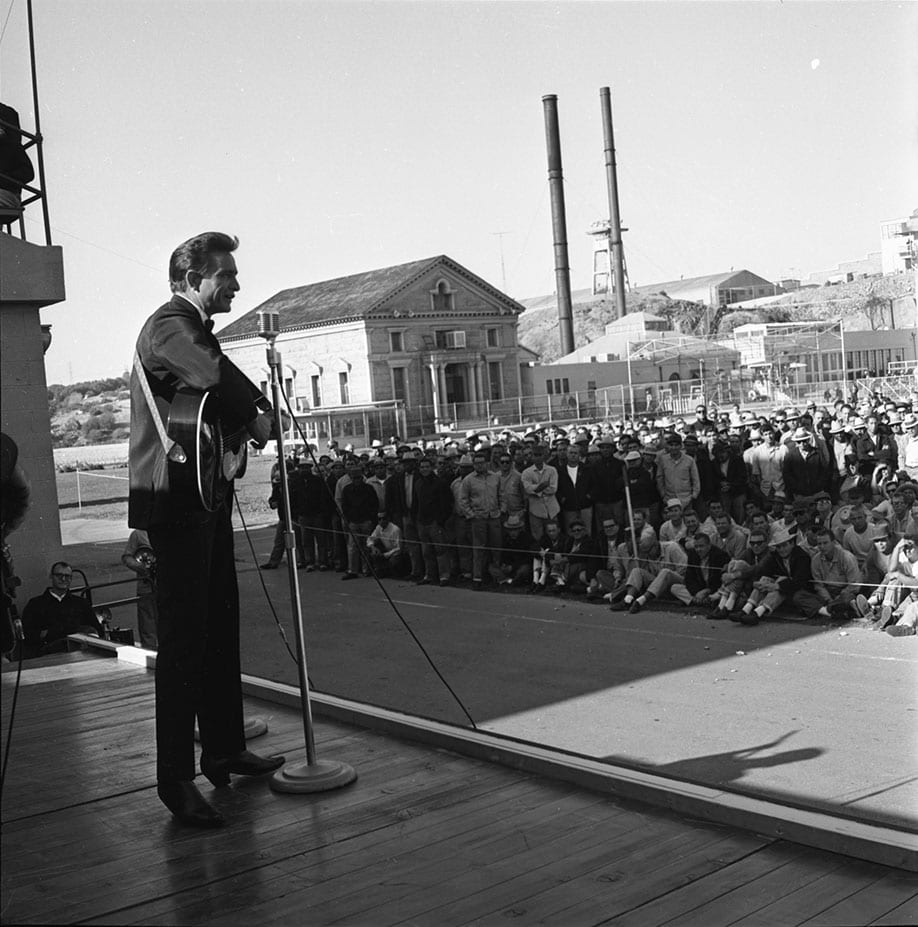This historical black-and-white photograph captures a mesmerizing musical performance set against an industrial backdrop. The central figure, who appears to be Johnny Cash, is clad in his signature black suit and dress shoes. He is holding a black guitar, strapped over his shoulder, and singing into an older style microphone reminiscent of the 1950s Elvis era, characterized by its distinctive design with a puffed front pointing upward.

Cash is performing on a slightly elevated stage with visible cables running off to the side, suggesting a technical setup. Off to the far side of the stage, a technical person is seated, ensuring the smooth operation of the show. Below the stage, the ground is covered with a mixture of dirt and gravel, upon which the audience is gathered.

The crowd, consisting predominantly of men dressed in similar attire, some possibly in work jackets and hats that could be hard hats, is seated and standing in a cleared-out area. A rope line in front of the stage holds back the enthusiastic audience, with several men sitting on the tarmac displaying a mixture of delight and amusement on their faces.

Behind the audience, the scene is framed by a chain-link fence and an assortment of industrial buildings. Dominating the background are two towering smokestacks, along with other large warehouse-like structures, reinforcing the industrial ambiance. To the right of the image, a slight reflection suggests that the photograph might have been taken through glass. The sky is indistinct, though it may be overcast, contributing to the nostalgic and historical feel of the photograph.